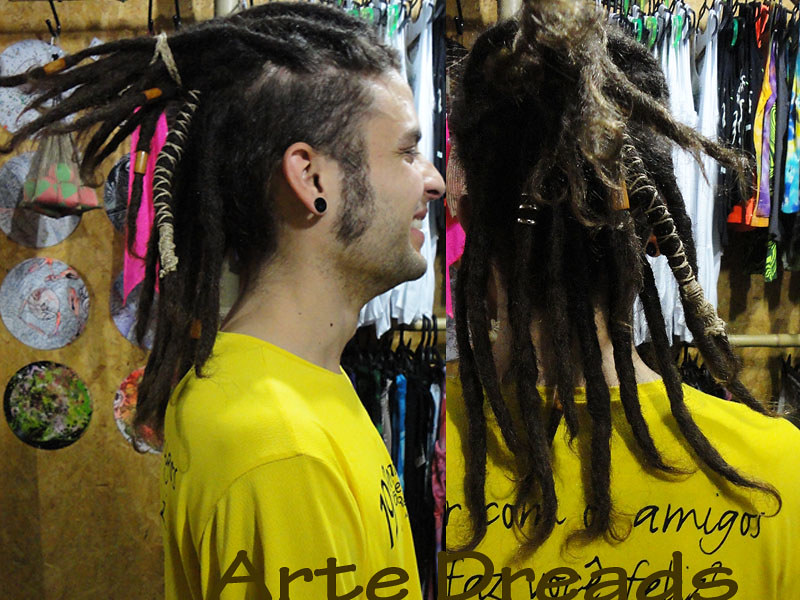The image features two photographs of the same man, labeled "Arte Dreads" at the bottom. The left photograph captures a side profile of the man, who is smiling and wearing a yellow t-shirt. His hair is styled in intricate dreadlocks, adorned with ribbons, including a noticeable pink one, and he has large black earrings and long sideburns. The right photograph shows the back of the man, revealing more details of his dreadlocks and the word "Amigos" printed in black on the back of his yellow shirt. The background includes a rack of clothing, displaying a variety of garments in colors such as white and multicolored, suggesting a store or closet-like setting. The combined image highlights the man's hairstyle from different angles, emphasizing the vibrant and eclectic nature of his dreadlocks and attire.